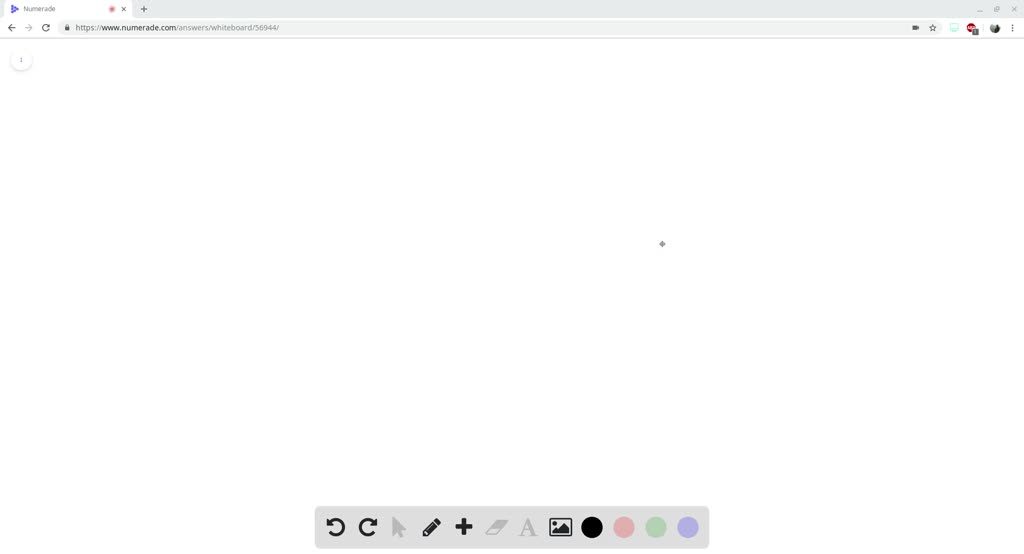Screenshot of the Numeraid Website: Interactive Online Whiteboard

This image is a screenshot of a webpage from the Numeraid website, accessible at www.numeraid.com. The highlighted section of the site is dedicated to their "answers/whiteboard" feature. The primary focus of this page is to provide an interactive, virtual whiteboard designed for users to draw, illustrate points, and jot down information as needed.

The interface prominently showcases a vast, white blank canvas that mimics a traditional whiteboard, allowing for freehand drawing and sketching. Along the bottom edge of the whiteboard area, a toolbar is visible, housing several essential options. These include undo and redo buttons, color selection tools offering a palette of colors such as black, red, green, and blue, and an eraser function. Additional features are different font styles and sizes to accommodate various writing and drawing needs. This comprehensive set of tools ensures that users can effectively communicate their ideas visually.

The screenshot captures a dynamic and versatile online tool aimed at facilitating information sharing and illustrative collaboration.